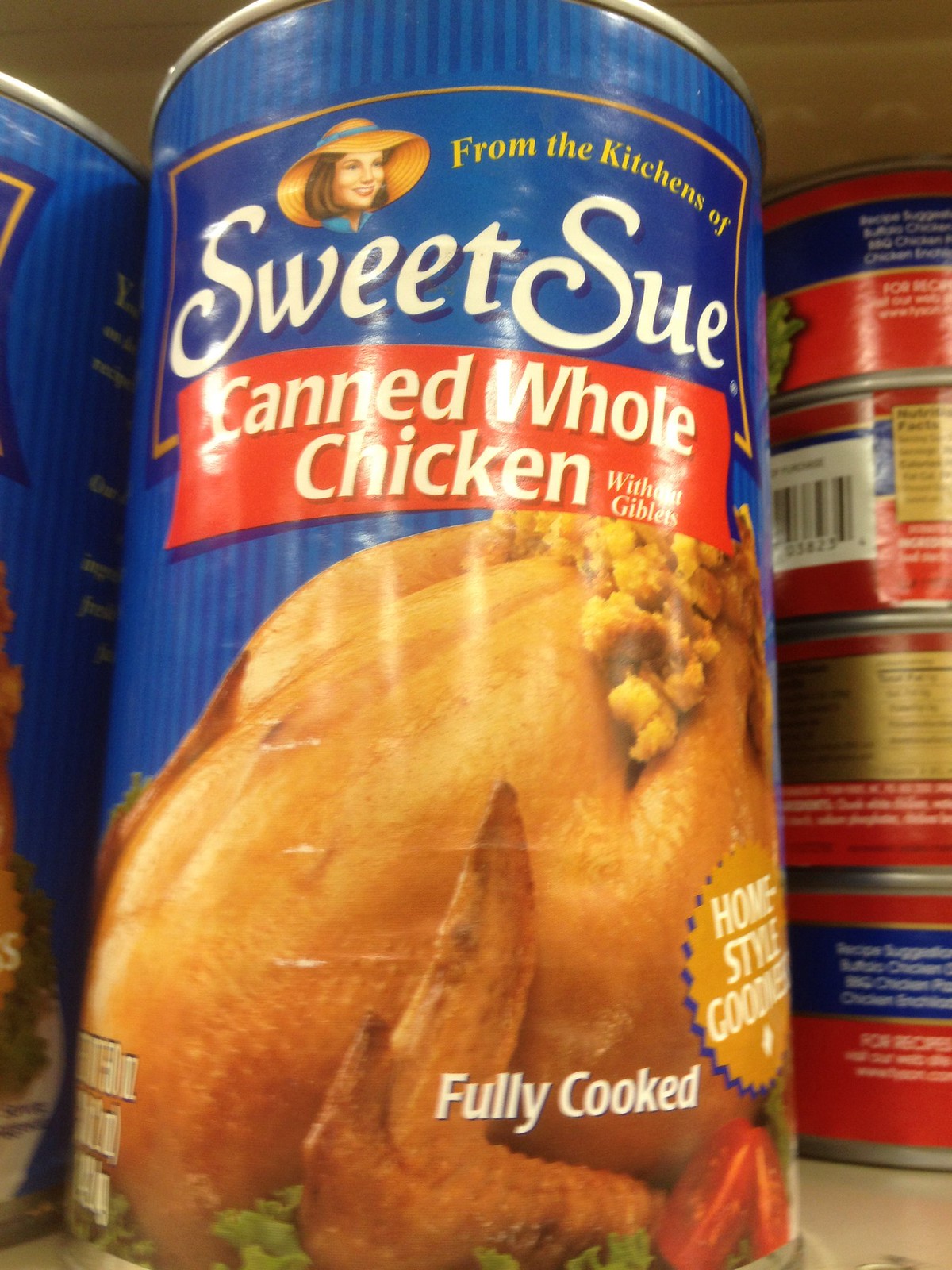This image features a prominently displayed blue can in the foreground, labeled "Sweet Sue." The label has a detailed design, with the name "Sweet Sue" written in bold white letters accompanied by a smiling woman’s face above it. The woman is wearing a straw hat and has chin-length brown hair. Situated to the right of the woman's face, the text "From the kitchens of" is written above the "Sweet Sue" name. Below "Sweet Sue," a red banner with white font reads "Canned Whole Chicken Without Giblets."

Further down, the label showcases a large, inviting image of a cooked chicken with stuffing placed on top of it. In smaller text at the bottom of the chicken image, the words "Fully Cooked" are clearly visible. Just below, a gold circle on the right-hand side of the can bears the inscription "Home Style Goodness." The text on the bottom left of the can's label is partially turned away and thus unreadable. The can is situated on a shelf surrounded by other various products, indicating that it is likely part of a grocery store display.